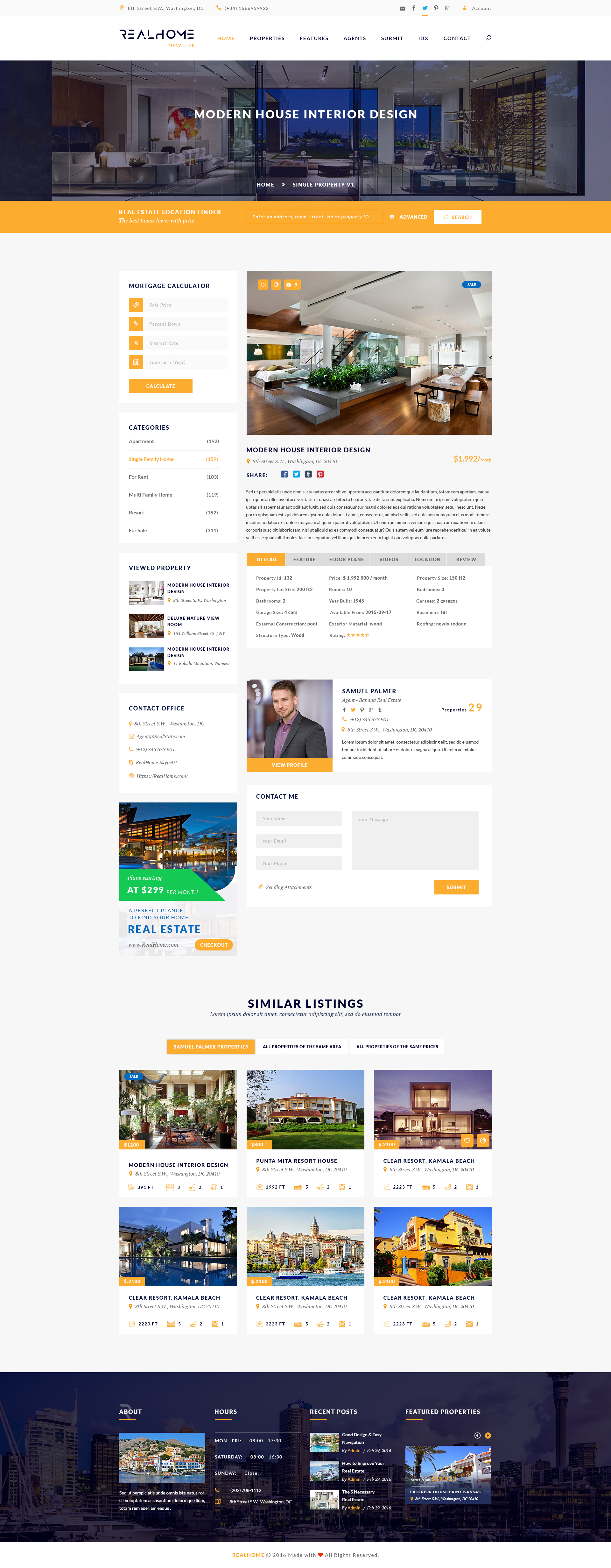This is an expansive screenshot of the Real Home website. The site title is displayed in a subtle gray at the upper left corner on a white background. Some of the smaller text throughout the site is extremely tiny and hard to read. 

To the right, an orange tab catches the eye, followed by a horizontal menu bar featuring five black tabs. At the top right, recognizable social media icons for Facebook and Twitter are visible.

Below these icons is a wide image banner with an orange border at the bottom. Prominent white text in the center declares "Modern House Interior Design," set against a faint background image of an ultra-modern luxury home overlooking the ocean. On the right side of the orange border, a white rectangular button, inscribed with orange text, provides a call to action, although the text is too small to read.

On the left, a column titled "Mortgage Calculator" in bold black text features four square buttons with labels and one larger orange button at the bottom, all with illegible text. Beneath this is a "Category" section, listing items in black and accompanied by numbers on the right, though the details are difficult to discern. 

Further down under "Viewed Property," three bold black headings align with small rectangular thumbnails on the left. The contact information for the office, contained within a "Contact Office" area, comprises six lines of indecipherable black text.

On the right-hand side, an advertisement displays an image of a well-lit building by a waterway with a green banner, listing the price at $2.99. "Real Estate" is emphasized in bold blue text below it.

An image above this advertisement showcases another luxurious modern home, accompanied by the bolded label "Modern House Interior Design." A "Share" button and icons for Facebook, Twitter, and two unfamiliar platforms are nearby. Light orange text in the upper right indicates a price, which is difficult to read, alongside an unreadable paragraph in black. 

Beneath the paragraph is a menu bar with five labels—the first white on orange, the other four black on gray. Further down are three columns of six lines of text each, all too small to read.

In a lower section, a white area features the name "Samuel Palmer" in bold with an image of a man in his late 30s on the left, underlined by an orange banner. The phrase "Contact Me" appears in bold black, followed by four gray text fields with tiny, unreadable text.

The "Similar Listings" section showcases two rows of three high-end, modern luxury homes. The top row includes "Modern House Interior Design," "Punta Meta Resort House," and "Clear Resort Kamala Beach." The bottom row repeats "Clear Resort Kamala Beach" for all three entries.

Finally, the bottom of the page has a thick black banner with four bold white sections labeled "About," "Hours," "Recent Post," and "Featured Properties." Accompanying these sections is a series of smaller white texts and several pictures of luxury homes, providing additional content.